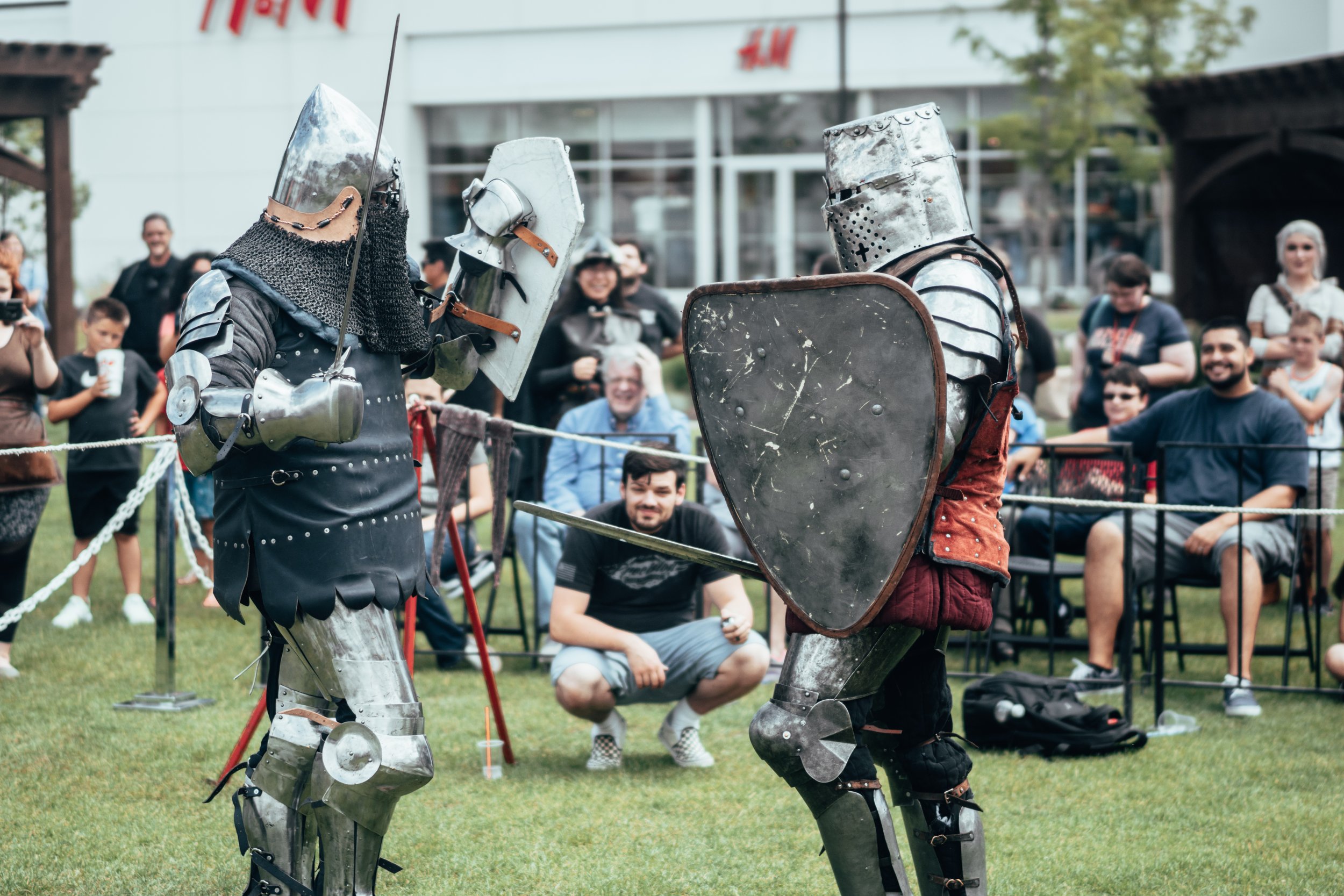The image captures an immersive medieval reenactment scene occurring outside an H&M store. In the foreground, two individuals are engaged in combat, dressed in elaborate medieval knight costumes. Their attire includes shiny silver armor and traditional, silver kettle helmets, reminiscent of the classic knight imagery. The knight on the right has a helmet featuring an etched cross, obscuring his face entirely. Both combatants are wielding thin, silver swords and brandishing shields, locked in a dramatic pose indicative of an intense duel.

In the background, a group of spectators is gathered behind a protective barrier, clad in modern-day attire. Some members of the audience are seated in chairs, while others stand, intently observing the spectacle. A man is squatting on the grass, engrossed in the action, with a plastic cup and an orange straw placed beside him. Near him, a backpack and an empty cup lie on the ground, adding to the scene's casual ambiance.

Among the spectators, a few individuals are captured filming the event, further emphasizing the blend of medieval and contemporary worlds. The H&M store's windows provide a stark contrast to the historical theme, situating this lively reenactment in an urban setting. The scene perfectly juxtaposes the past with the present, creating a unique and engaging visual narrative.